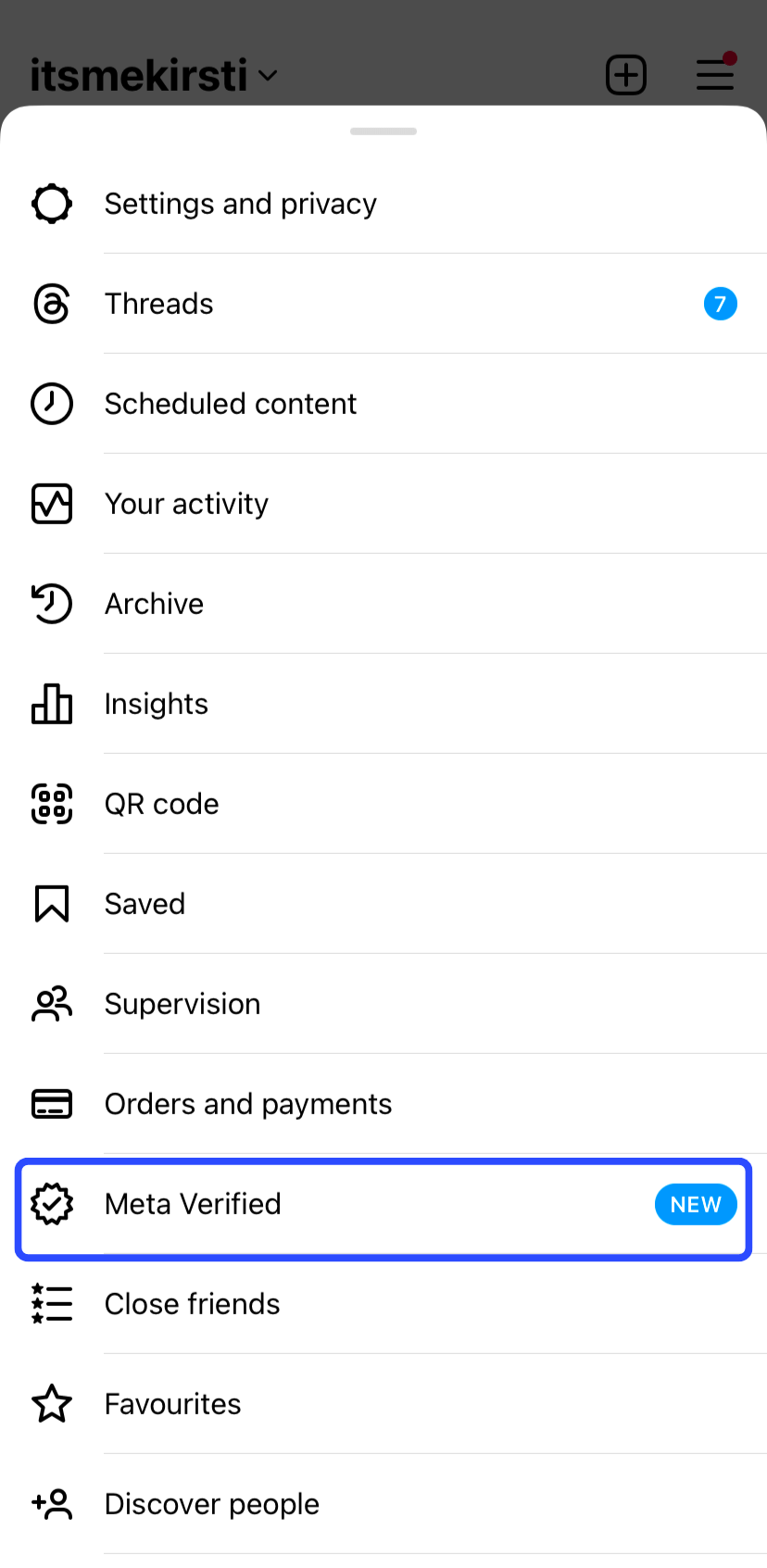This image is a screenshot showcasing a settings page with a variety of options listed in black text on a white background. At the top of the page, there is a heading, “Settings and Privacy,” accompanied by a circular gear icon. Below this heading, there is an organized list of options, each with its own icon for easy identification:

1. **Threads** – Displayed with an “@” handle.
2. **Scheduled Content** – Identified by a clock icon.
3. **Your Activity** – Represented by a bar graph icon.
4. **Archive** – Illustrated with a clock and backward arrow icon.
5. **Insights** – Marked by a bar graph icon.
6. **QR Code** – Showcased with an image of a QR code.
7. **Saved** – Denoted by a bookmark icon.
8. **Supervision** – Highlighted by the outline of two people.
9. **Orders and Payments** – Signified by the outline of a credit card.
10. **Meta Verified** – Distinguished by a circular badge with a check mark at the center, enclosed in a blue box to draw attention.
11. **Close Friends** – An additional section without a specific icon mentioned.
12. **Favorites** – Indicated by a star outline.
13. **Discover People** – Presented as a button.

Each of these options is designed to provide a specific function, enhancing the user’s ability to manage their account effectively through this comprehensive settings page.